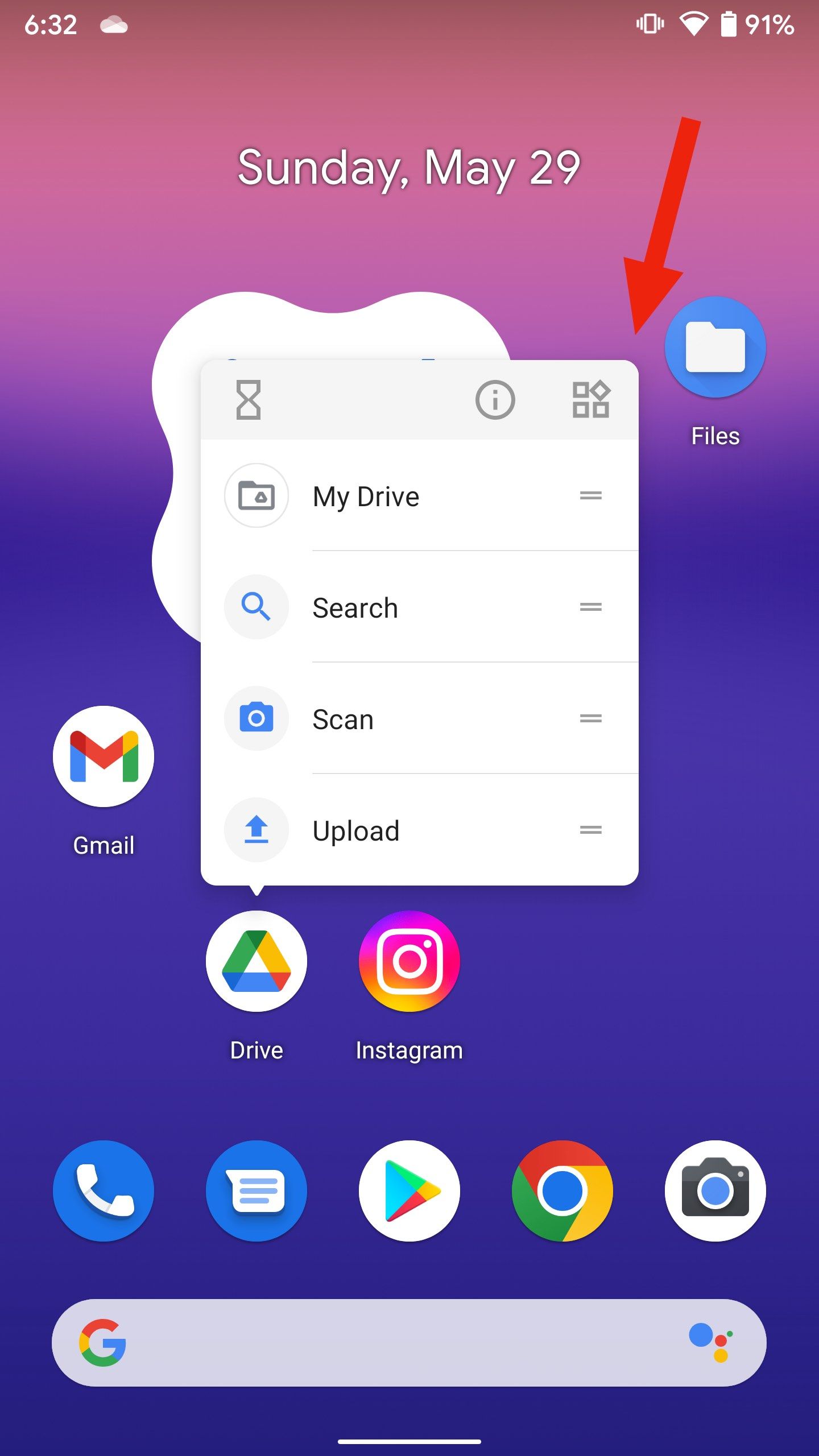This image is a close-up screenshot of a phone’s home screen, highlighting the Google Drive app through a detailed pop-up information box. The pop-up is a white square with a small triangle at the bottom, pointing directly at the Google Drive app to indicate focus. 

The pop-up consists of various elements arranged from top to bottom. Starting at the top, there is a row of icons including an hourglass symbol on the left, followed by an eye icon encased in a circle, and then a grid of four squares on the right side of the row. Below these icons, a list of options is displayed, each accompanied by a corresponding icon:
1. **My Drive** - Likely represented by an appropriate Google Drive emblem.
2. **Search** - Accompanied by a magnifying glass icon.
3. **Scan** - Indicated by a camera or scanner icon.
4. **Upload** - Marked by an upward arrow symbol, typical of upload functionalities.

Each item in the list is followed by two horizontal lines, possibly indicating further details or options available by selecting each item.

Additionally, the phone's home screen itself has a prominent red arrow originating from the top-right corner, pointing downward towards the corner of the pop-up box, emphasizing the focal point of the screenshot.

The background of the home screen showcases a visually appealing gradient starting with pink hues at the top gradually transitioning into purple towards the bottom. There are also various app icons visible on the home screen, including well-known applications such as Gmail, Instagram, and Facebook.